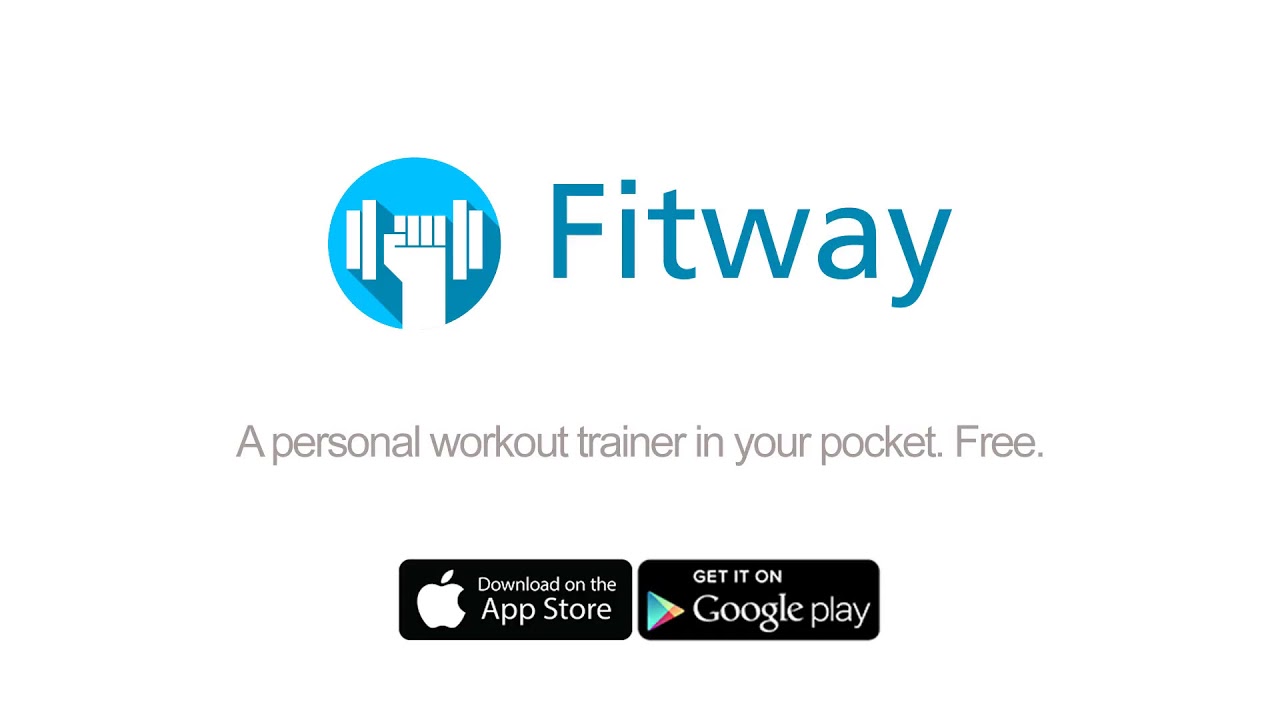The image is an advertisement for a fitness app named "Fitway" displayed on a completely white background. At the top left corner, there is a bright blue circular logo featuring a simplistic white hand holding a dumbbell, with the fingers and dumbbell depicted as blocky, rectangular shapes. To the right of this logo, the name "FITWAY" is prominently written in a large, bluish-gray font. Below this, in a slightly smaller gray font, the tagline reads, "A personal workout trainer in your pocket," followed by the word "FREE." Beneath this text, there are two wide black rectangles with curved corners. The left rectangle contains the Apple logo with the text "Download on the App Store" in white, while the right rectangle features the Google Play logo with a colorful triangle and the text "Get it on Google Play" in white.